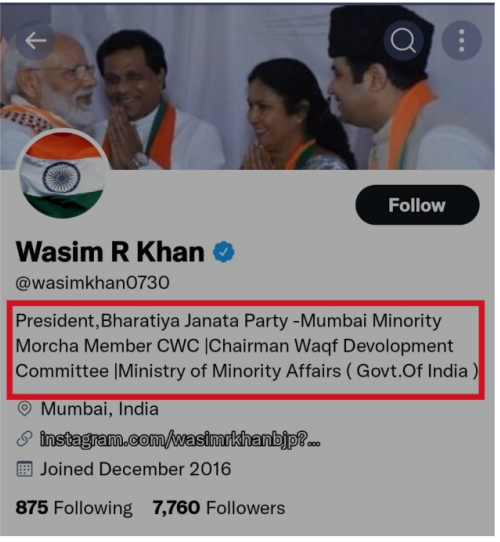**Caption:**
This image is a vertical, portrait-style screenshot of a Twitter account, showcasing a well-defined layout. At the very top, there's a photo depicting four individuals engaged in interaction. On the left, a man with glasses, a white beard, and dressed in white can be seen. Next to him stands another man, likely of Indian descent, with black hair, wearing white attire and an orange item draped over his shoulders. Beside him, a woman with brown hair and brown skin is present. The fourth person, a man with dark hair and possibly a dark fez, also dons white clothing complemented by an orange garment.

Moving down, the profile picture of the account is the Indian flag. The account name is "Wasim R. Khan," verified with a blue check mark, and the Twitter handle is @WasimKhan0730. Positioned to the right is a black "Follow" button.

In the bio section, the description reads: "President Bharatiya Janata Party, Mumbai Minority, Merchant Members CWC, Chairman WAQF Development Committee, Ministry of Minority Affairs (Government of India)." This text is enclosed within a red rectangle, making the essential information easily noticeable.